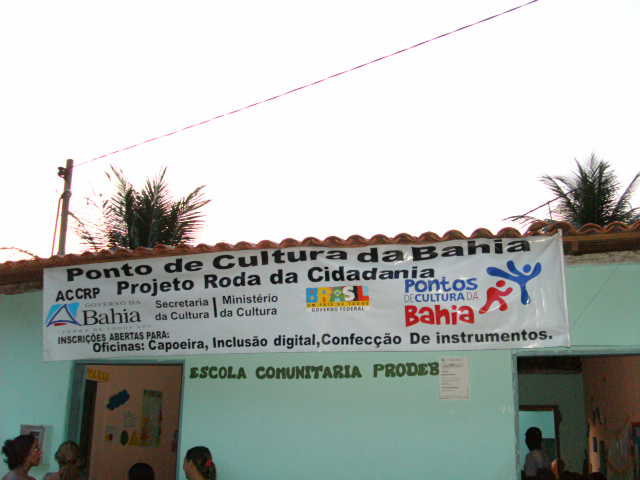This outdoor daytime photograph captures a light greenish-blue, smooth-faced community center or storefront with a flat façade, slightly wider than it is tall. The building's red clay tile roof supports a white banner that hangs down, displaying "Ponto de Cultura de Bahia, Projeto Roda da Cidade" in black print, along with several sponsor logos. Below, on the left side, a brown door is flanked by people gathered, seemingly waiting to enter. Adjacent to the door, "Escola Comunitaria Prode..." is written in green print on the outer wall, though the text is partially obscured by a white piece of paper. The building's right side features an open hallway. Above the roof, a featureless, whited-out sky is framed by two palm trees and interrupted by a single utility pole with a wire extending towards the photograph's upper right.